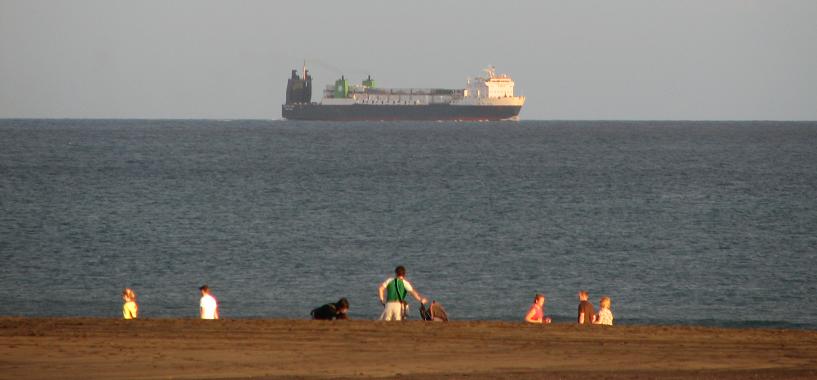In this detailed image, we see a bustling beachfront scene set in the middle of the day. The sandy beach at the bottom of the image stretches out with a light brown hue, dotted with six distinct people. To the left, a man and woman walk together; the man is in a dark shirt, while the woman dons a yellow top. In the center stands a man in a green shirt with white sleeves and tan shorts, his gaze fixed on the large cargo ship offshore. The ship, dominating the horizon where the deep blue sea meets the sky, features a striking dark hull with a red stripe and white cargo bins stacked mid-deck. On the right side of the beach, a group of three people engage in a discussion: a woman in a red or pink tank top, a man in a dark shirt, and another woman in white. The vast body of water takes up the central part of the image, reflecting the clear blue sky overhead, while the ship, sizable and imposing, floats serenely near the top of the frame. The vivid colors of brown, white, yellow, green, pink, blue, and gray paint a lively outdoor scene.